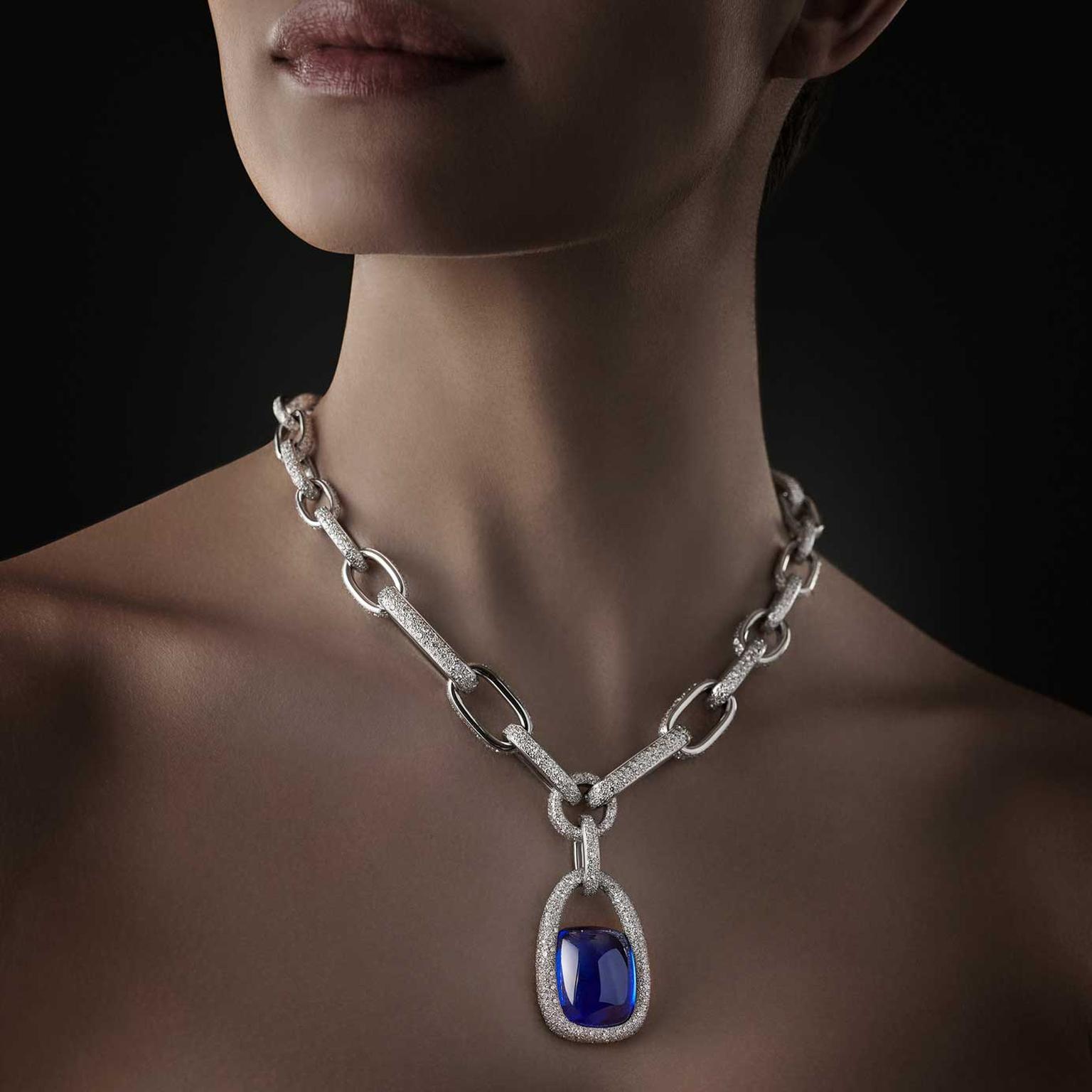This professional product photograph features a close-up of a female model on a black background, expertly showcasing a luxurious, statement silver necklace. The model's face is mostly cropped out, focusing on her elegantly long neck, collarbones, and the top of her chest, alongside her collarbones and lips adorned with light-colored lipstick. The airbrushed, blemish-free skin adds to the high-end feel of the image, resembling a luxury brand advertisement.

The necklace itself consists of thick, chunky chain links, alternating between shiny silver and intricately designed sections, lending an opulent texture to the piece. The focal point is a large, oval-shaped pendant framed by the chain, featuring a stunning, multifaceted blue stone that transitions from a deep sapphire hue in the center to lighter, reflective shades on the edges. The minimalist, dark background and subtle lighting emphasize the necklace, making it the central element of the photograph. The overall dim ambiance, with just a hint of light from the left, creates a dramatic and elegant presentation, underlining the necklace's sophistication and desirability.